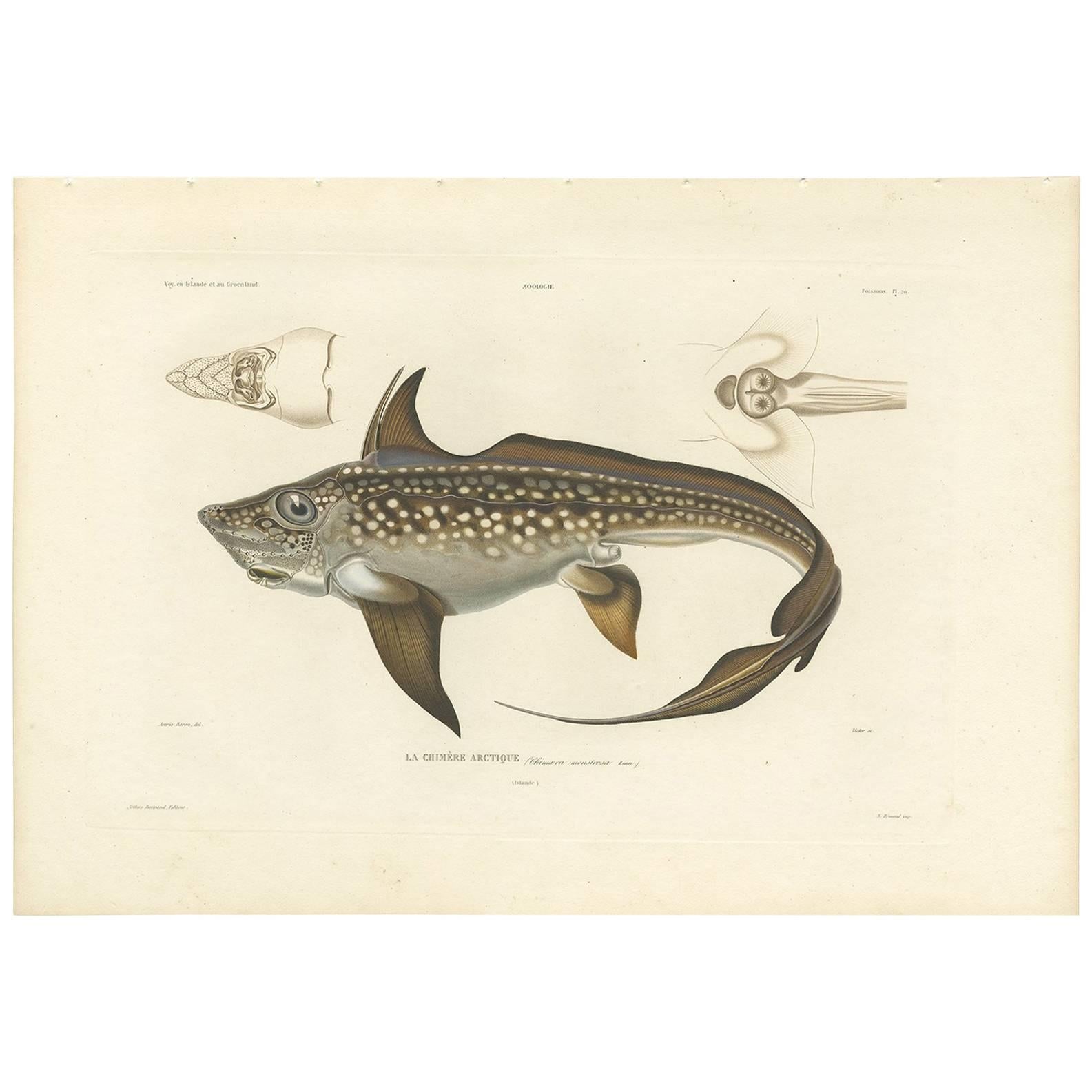The image depicts a detailed, vintage-style illustration of a fish, set against a faded beige background resembling old textbook pages. The fish itself has a brownish-gray coloration with white spots scattered across its back, and its white belly contrasts with the darker hues of its body. It features triangular-shaped fins on both the top and bottom, and a large, curved tail. The illustration shows the fish facing left, with its eye clearly visible. Above the fish, thinly drawn lines suggest an x-ray view of its head, providing an intricate look at its internal structures. Additional diagrams to the upper right and left highlight specific parts of the fish’s anatomy, possibly bones or internal organs, and each cross-section shows intricate details with accompanying labels. Below the fish, in fine print, is the name of the species, adding a scholarly touch to the illustration. This detailed diagram has the appearance of being taken from an old scientific book or archival material.